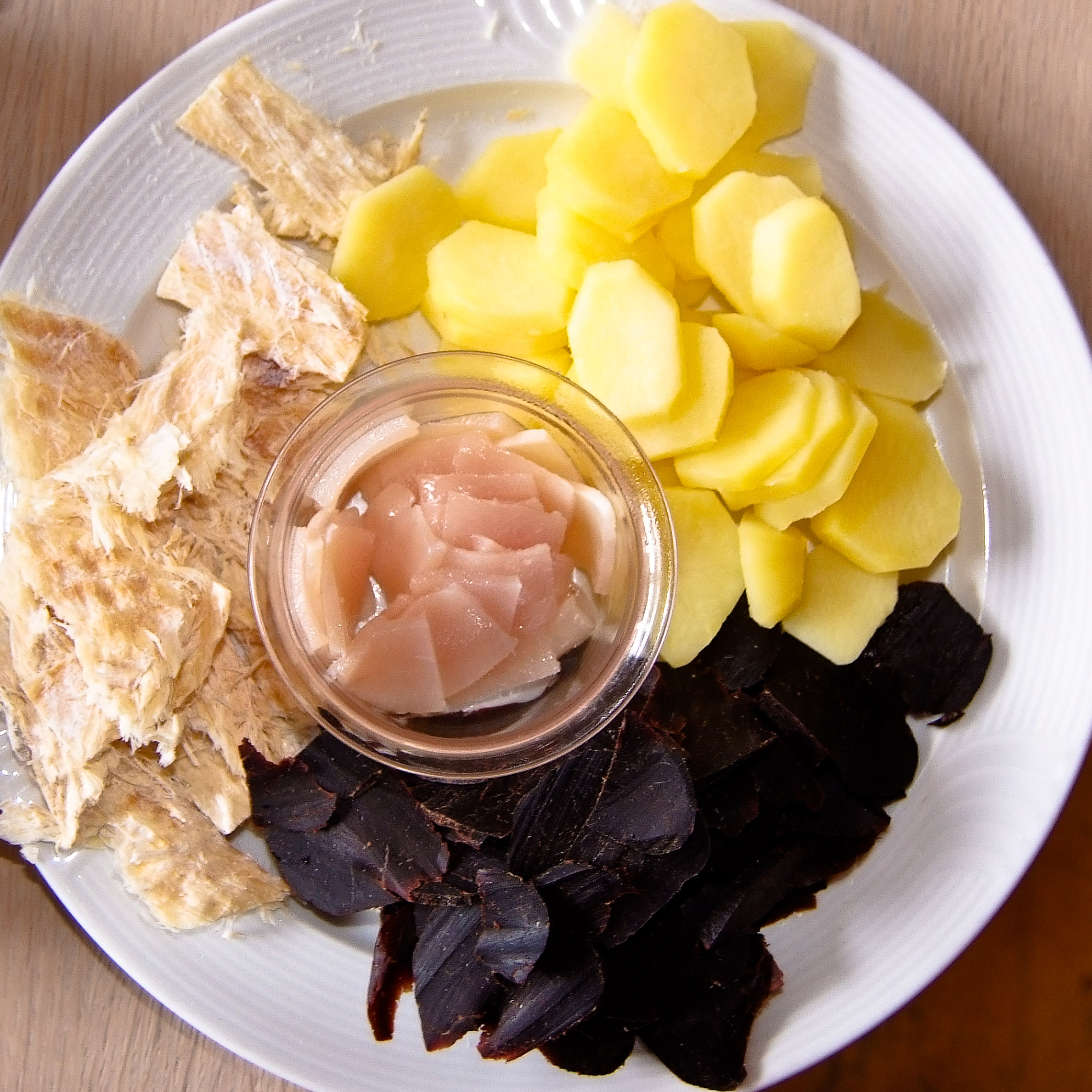The image depicts a detailed and meticulously arranged dish set on a white circular ceramic plate with an engraved textured border. The plate sits on a wooden table, the pale pine-colored surface barely visible due to the close-up nature of the photo. At the center of the plate is a small, clear glass bowl containing thinly sliced raw meat, possibly resembling smoked salmon or ceviche-style chicken, suspended in a liquid.

The surrounding plate features a variety of foods: on the upper right corner are neatly peeled, small hexagon-shaped potato pieces with a yellow hue, likely Yukon potatoes. The bottom section contains dark, almost beef jerky-like strips, which might be a form of dried or cured meat such as beef or darkly colored truffle shavings. To the left, there's a pile of cracker-like bread, possibly broken-up crusts or a pale beige substance like cassava.

The dish's color palette includes shades of beige, golden yellow, and deep dark purple, contributing to an overall visual contrast on the white ceramic background. The arrangement appears to be very deliberate, akin to a traditional charcuterie board, intended for tasting and mixing different flavors and textures together.